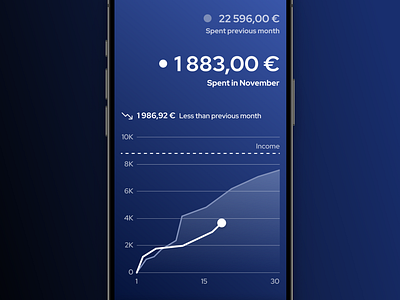The image depicts a smartphone screen with a distinctly dark blue background that transitions into a lighter shade. On the screen, white text displays detailed financial data related to stock performance. At the top right corner, the figure "22,596.00 euros" is prominently featured. Below this, it states, "Sprint previous month" followed by "1883.00 E" in a white circle, indicating the amount spent in November, with "1986.92 E less than previous month" further detailed underneath. 

The screen also includes two line graphs—one white and one blue—illustrating the stock's performance metrics. The white graph rises slightly and terminates at a marked white circle near the "4k" point on the Y-axis. The X-axis and Y-axis are labeled with numeric values and income figures, respectively, both showing upward trends. All this information stands out against the blue-toned background of the smartphone display.